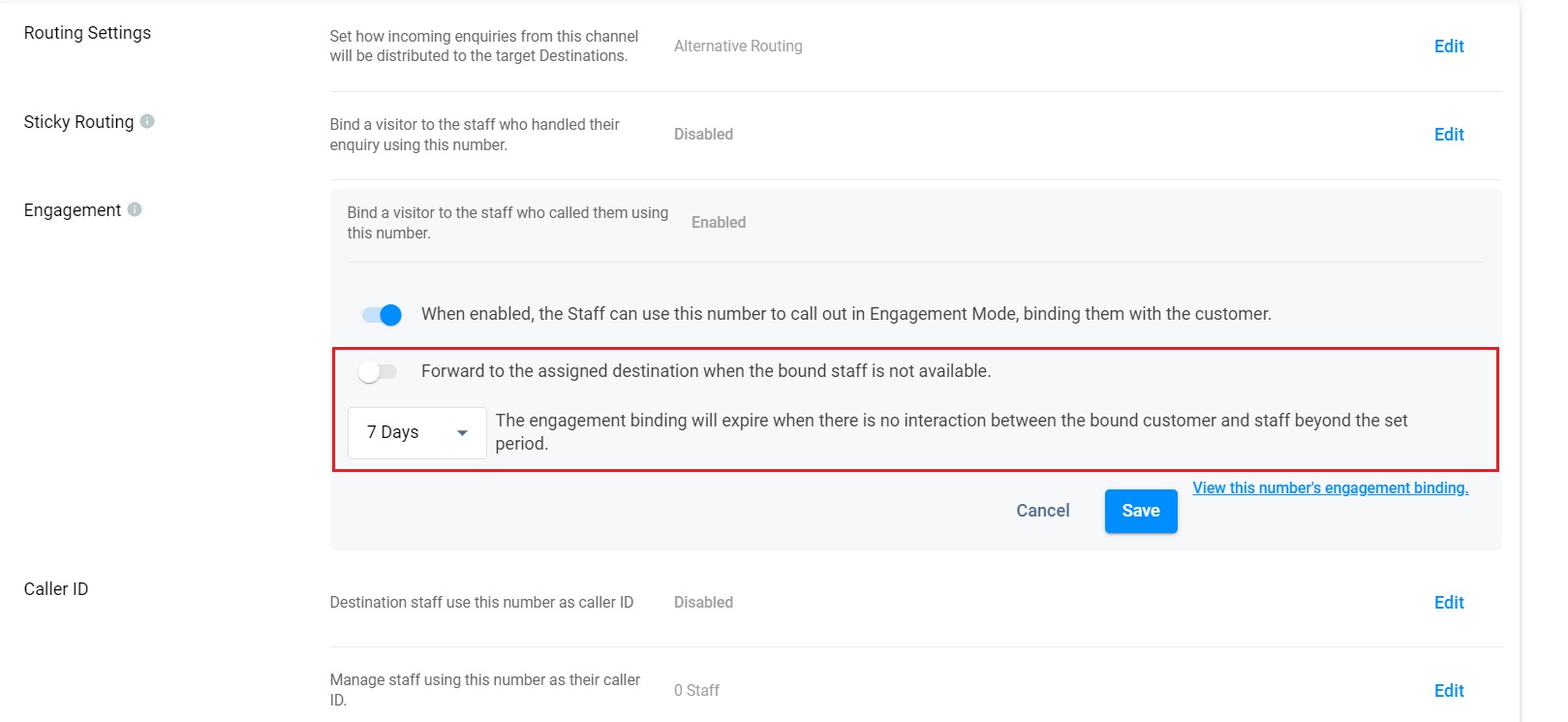This image depicts a detailed interface for managing routing settings, likely utilized by a call center or an outbound marketing team. The interface is divided into several sections, each accompanied by edit buttons for customization.

On the upper left, under "Routing Settings," users are instructed to define how many incoming inquiries from a specified channel will be distributed to target destinations. Below this, there's a setting for "Alternative Routing," with an edit button adjacent to it, allowing further configuration.

Further down, a section labeled "Sticky Routing" features a notable exclamation icon. This section details an option to bind a visitor to the staff member who initially handled their inquiry using a specific number, but it is currently disabled. An edit button is present for enabling or adjusting this feature.

As we progress towards the middle of the interface, the "Engagement" section is highlighted, also marked with an exclamation icon. This setting, which is currently enabled, indicates that a visitor will be connected to the staff member who called them using a given number. Beneath this, an additional option states that when enabled, staff can use this number to call out in engagement mode, binding them with the customer. This option is indicated to be active via a blue slider.

Another section outlines the forwarding of calls to an assigned destination if the bound staff member is unavailable. This setting appears to be inactive and specifies that the engagement binding will expire if there is no interaction between the customer and the staff member within a set period of seven days. This section is notably outlined with a red rectangular border, suggesting its importance.

At the interface's bottom, there is a "Caller ID" configuration option. It states that destination staff can use this number as a caller ID, but this feature is currently disabled. Additionally, it mentions the option to manage which staff members are authorized to use this number as their caller ID, currently set to zero staff.

Each section is equipped with edit buttons, allowing for detailed customization. The interface concludes with options to save or cancel any changes made. This setup is indicative of a sophisticated system designed for routing and managing calls efficiently, essential for operations in a call center or a sales and marketing environment.